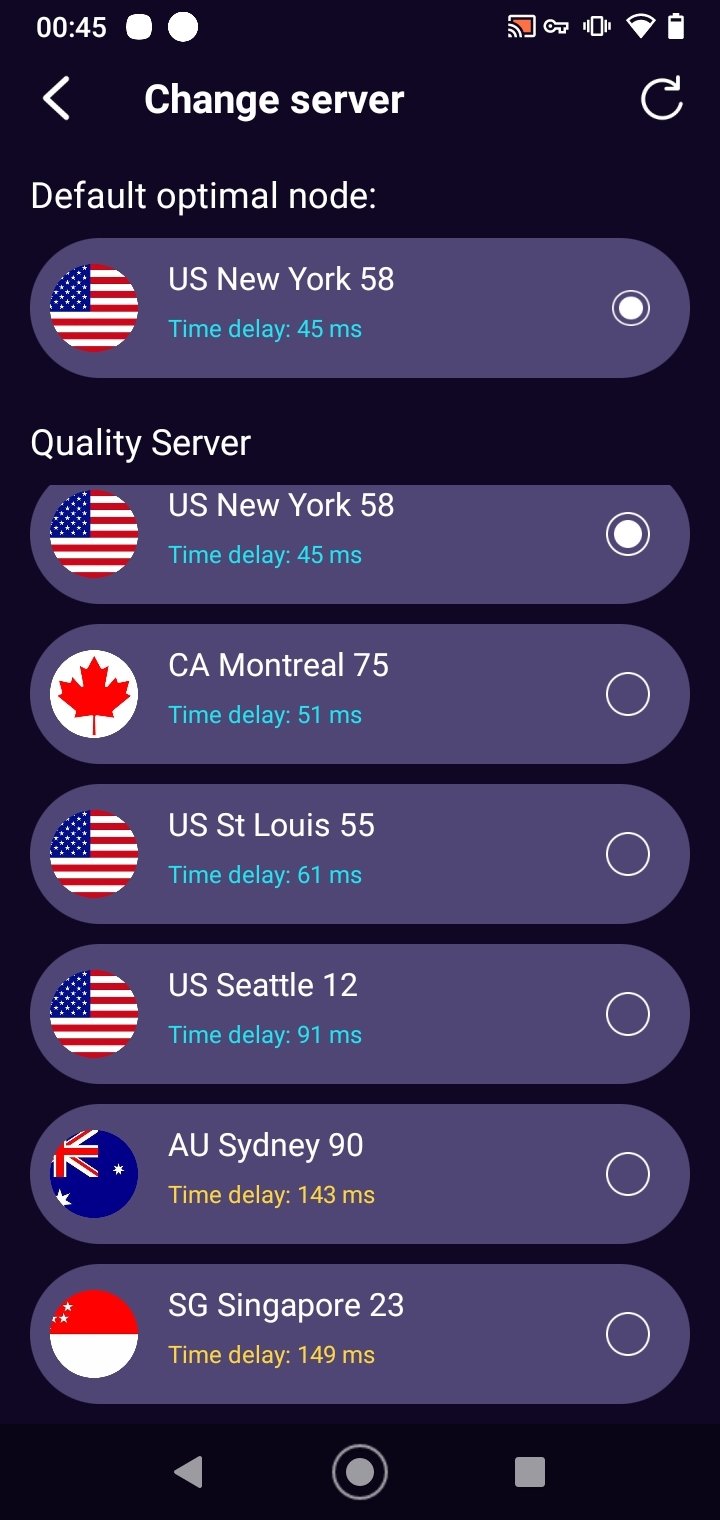This screenshot is captured from a cell phone featuring a vertical rectangular display. At the top left corner, the notation reads "45 seconds," indicating the duration of the current session or action. On the right-hand side, the signal strength indicator shows a red bar, suggesting very low or poor signal reception.

The main content of the screen pertains to the "Change Server" function, likely for a VPN application. This interface contains several options presented in purple elongated ovals. The first option is labeled "Default Optimal Mode," and beneath it, there is a detailed option labeled "U.S. New York 58" accompanied by a time delay marker. Below that header, in black text, the term "Quality Server" appears, also offering the "U.S. New York" option, with both selections highlighted in purple ovals on the right side.

Additional server options listed are Montreal, St. Louis, Seattle, Sydney, and Singapore, each represented in a similar purple oval format. The image seems to show someone actively trying to change their VPN server on their cell phone to optimize their online security or connectivity.